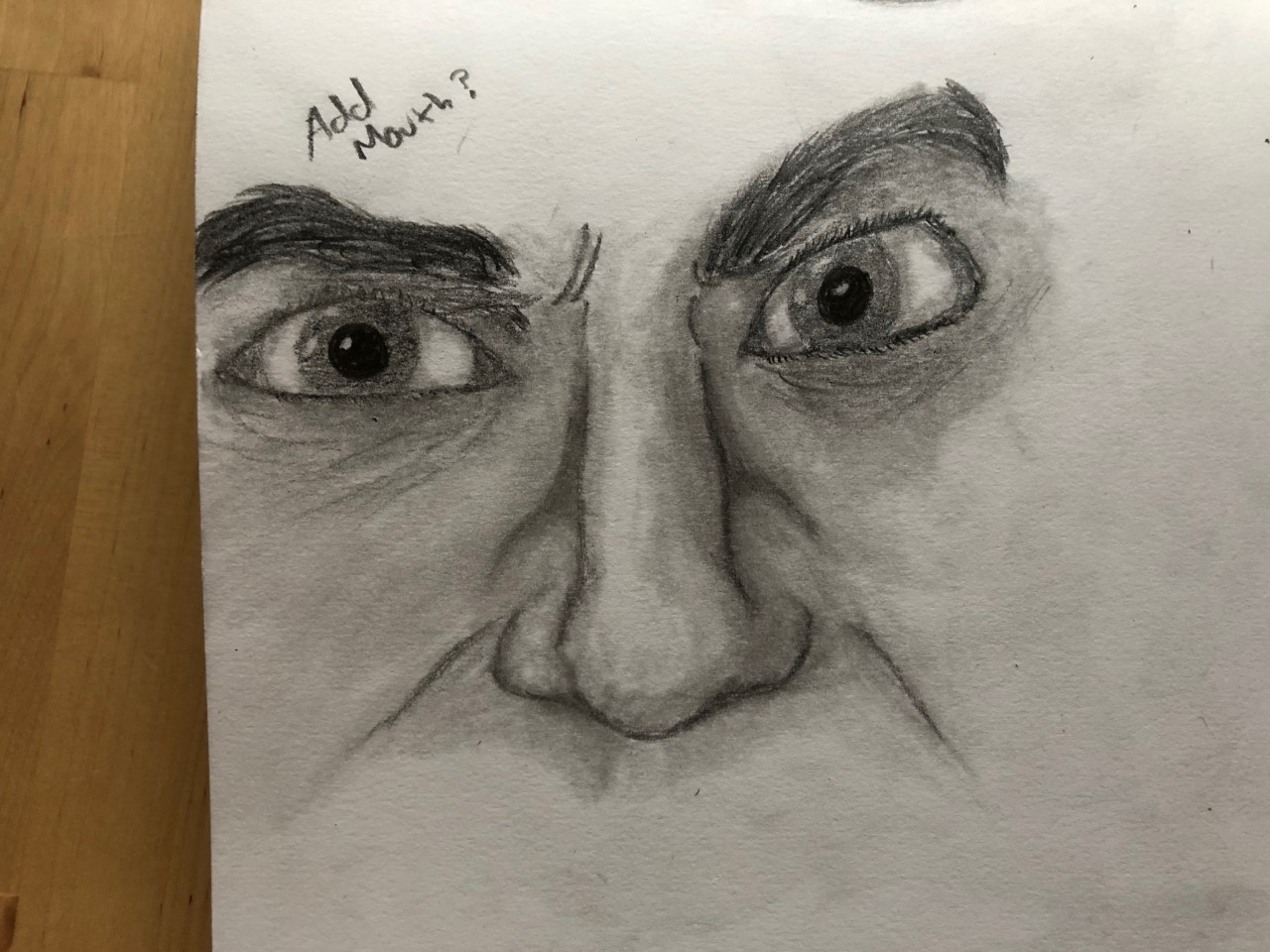The image depicts a highly detailed, black-and-white charcoal sketch focused on the central portion of a face, prominently featuring expressive eyes, a defined nose, and bushy eyebrows. The sketch employs various shades of gray to add depth and realism, particularly around the eyes and nose. The pupils are gray, and the eyelashes are short. The face shows intricate lines suggesting expression, especially near the top of the nose, indicating a slight scrunch. Notably, there is no mouth drawn; instead, above the left eyebrow, the phrase "add mouth?" is written in black text. The sketch resides on a light gray canvas, partially resting on a brown wooden table visible on the left side of the image.